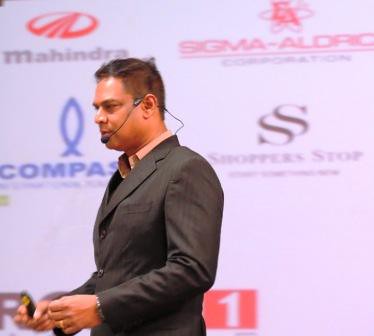The image depicts a well-dressed man, likely in his forties, wearing a gray suit jacket over a peach or orange shirt. He has a silver watch on his wrist and a ring on one of his fingers. The man is captured in a side view, facing left, as he appears to be speaking through a gray headpiece with an attached microphone. His hands are positioned in front of him, and he might be holding a clicker for changing presentation slides. The background is predominantly white, featuring several prominent logos and text. The logos include "Sigma-Aldrich Corporation," "Mahindra" with a red emblem above it, "Compass" accompanied by a sideways fish logo, and "Shoppers Stop." A red number 1 is also visible on the backdrop. The setting suggests that the man is in the middle of delivering a presentation at a corporate event or seminar.